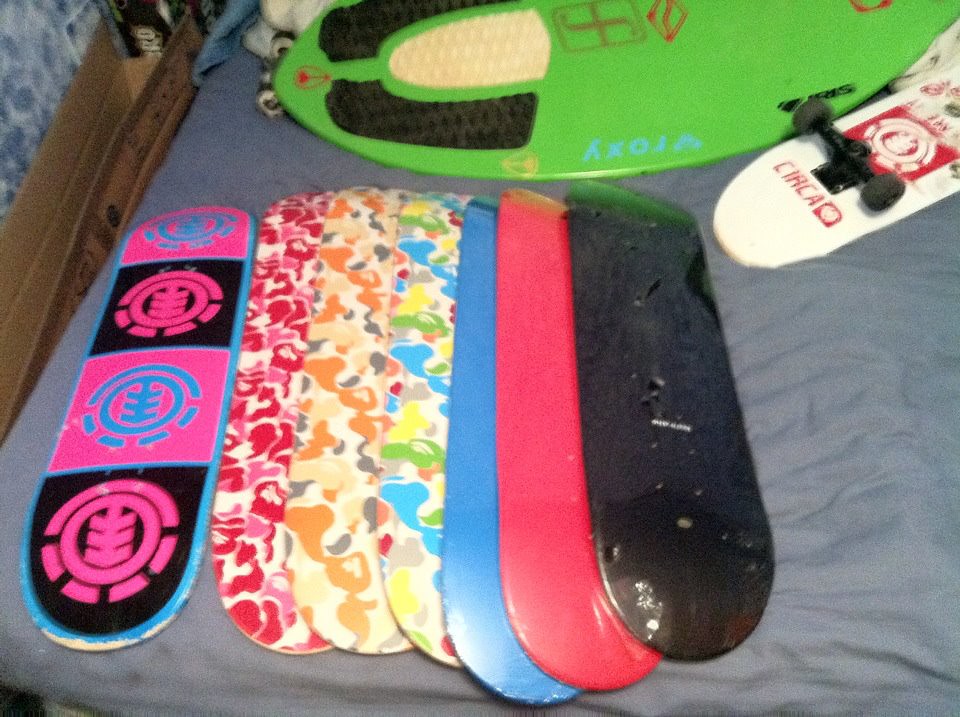This image is a top-down photograph of a bed covered with several skateboards, accompanied by distinctive blue wallpaper on the left-hand side of the frame. The blue sheet on the bed is slightly crumpled. At the top of the bed, from left to right, are two skateboards with wheels: one is green with black and red designs, while another is white with "CIACA" written in red letters and has black wheels. Towards the bottom left of the bed, a row of seven skateboards lies side by side, all without wheels. These include a skateboard with alternating pink and black squares, three adorned with floral-like patterns, and three solid-colored boards in blue, red, and black. Among the floral-patterned skateboards, one displays blue, green, yellow, and gray blotches; another features orange, tan, gray, and white splotches; while the other two have similar red, white, and pink blotches. Several of these skateboards exhibit a variety of colors and patterns, contributing to the diverse and somewhat chaotic appearance of the collection.